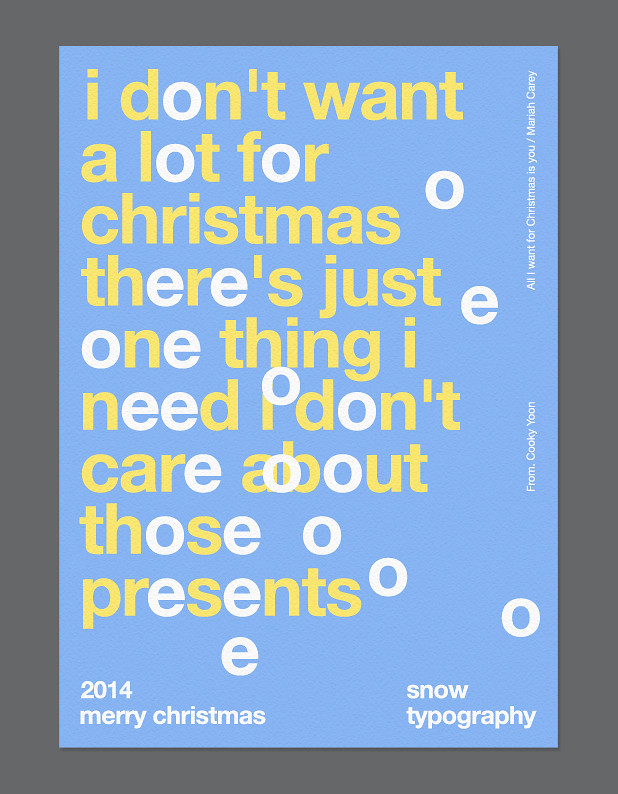The image in portrait view features a dark gray border framing a bright blue background adorned with white and yellow text. The text quotes a lyric from the song "All I Want for Christmas Is You" by Mariah Carey, reading: "I don't want a lot for Christmas, there's just one thing I need, I don't care about those presents." This cheerful message is presented in alternating white and yellow fonts. At the bottom of the image, the text "2014 Merry Christmas" is displayed in white on the left, while the bottom right corner features "snow typography." Along the right-hand side, it reads "from Kuki Yoon." The overall composition evokes a festive spirit, with the contrasting colors and fonts adding to the visual interest while timestamping the image to the 2014 holiday season.